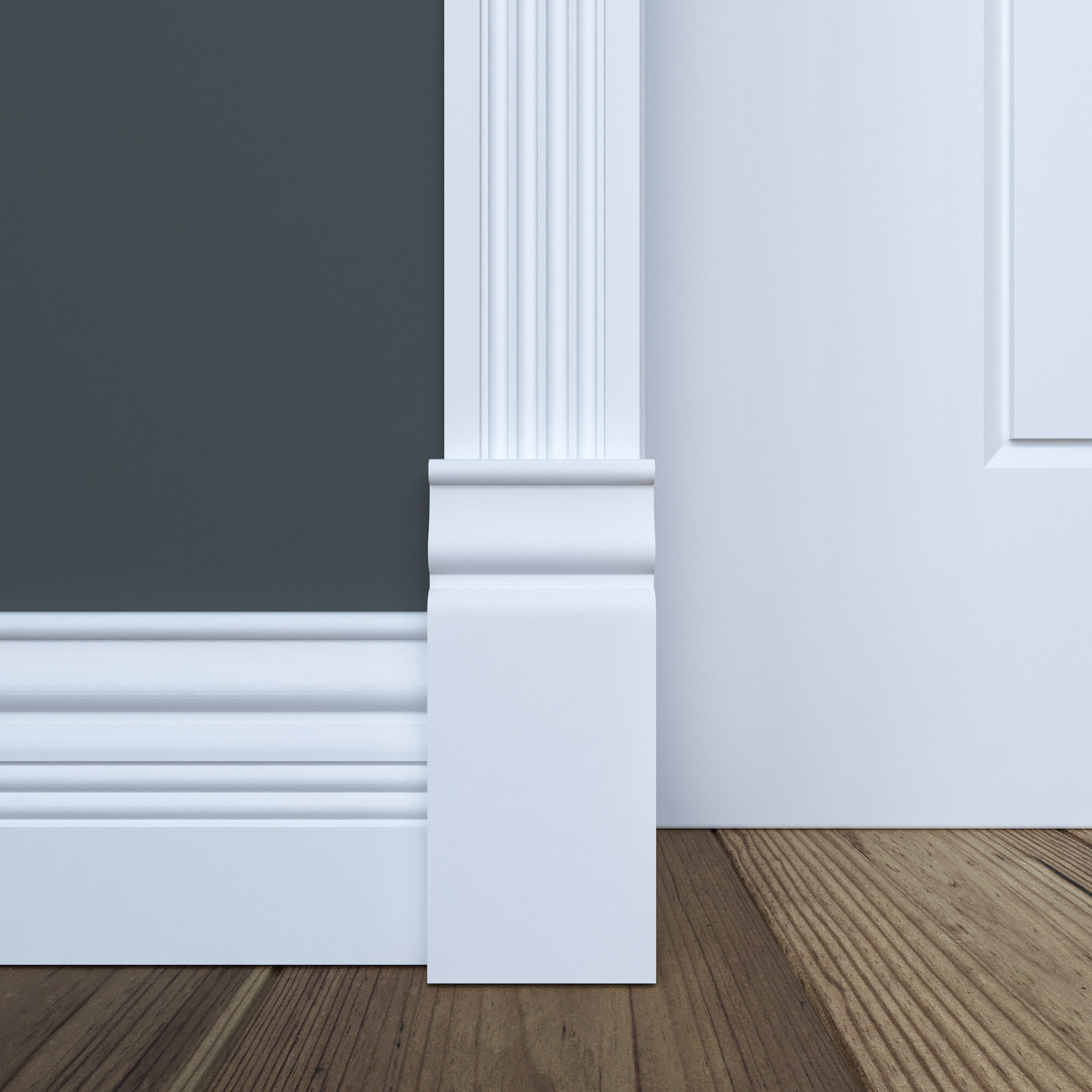The image presents a detailed, three-dimensional graphical rendering, focusing on a section of a room where a white-painted wall and a matching white pillar are prominently displayed. The pillar, situated against the wall and characterized by vertical lines running from its top to its base, is distinctly divided into two sections with a thicker middle layer. On the left side of the pillar, a gray part of the wall is noticeable. The floor, composed of fine brown wood, features intricate patterns where the wood converges, adding to the room’s aesthetic. To the right, additional lines and a rectangular pattern at the top right further contribute to the composition.